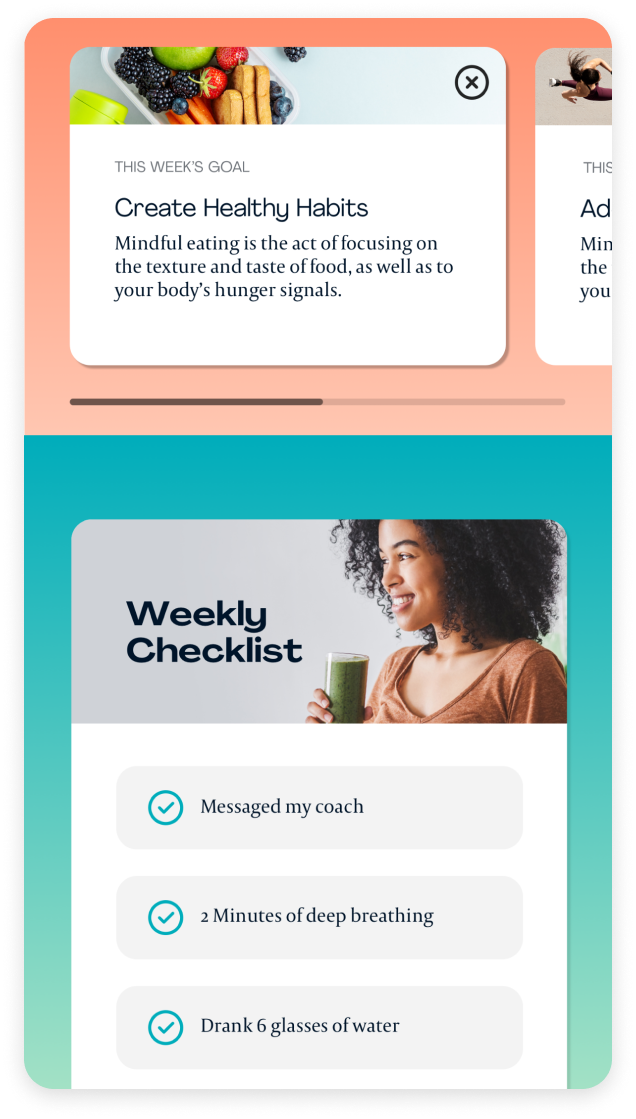A smartphone screen displays a detailed health and mindfulness application interface. At the top of the screen, there's a prominent red or pink square that showcases an assortment of berries and fruits against a gray background with an 'X' symbol. The screen features a text box on a white background containing the motivational phrase, "Create healthy habits: Mindful eating is the act of focusing on the texture and taste of food as well as your body's hunger signals."

Below this message is a blue bar that leads into a weekly checklist. A woman wearing a brown shirt is seen holding a glass filled with green juice. Further down, a message from the user's coach is displayed with several key points, each followed by a checkmark: "Two minutes of deep breathing," among other tasks. Finally, it includes a reminder to drink six glasses of water daily.

The entire interface is set against a consistent gray background, with various elements such as text, images, and checklists intricately integrated into the design. The overall intention of the interface is to promote mindfulness and healthy habits with a visually engaging and user-friendly presentation.